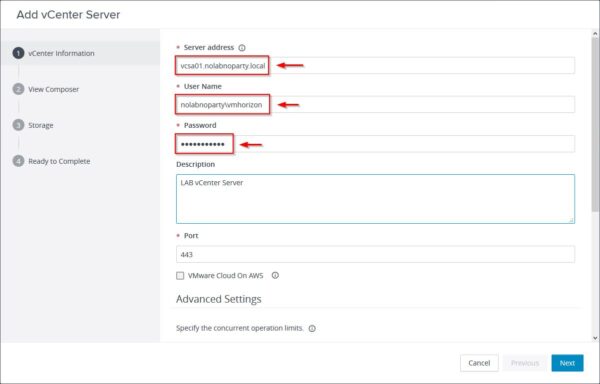The image showcases an application interface predominantly featuring white, black, and red colors. At the top of the screen, the words "Add," "vCenter," and "Server" are displayed in black font. Below this, there is a light gray panel with numbers indicating steps in a process. 

1. The first step is marked by a bold white number "1" inside a black circle and labeled as "vCenter Information."
2. The second step, connected by a line below, is a black circle with a white number "2," indicating "View Composer."
3. Continuing down, the third step is depicted with a black circle and a white number "3," labeled as "Storage."
4. The final step is marked by a black circle with a white number "4," indicating "Ready to Complete."

To the right on a white background, fields for entering server information are shown. There is a red box with a red arrow pointing left, labeled "vcsa01." The box also indicates "none," "no lab," and "no party.logo." Below this, a field for "Username" is also highlighted in a similar red box with a red arrow.